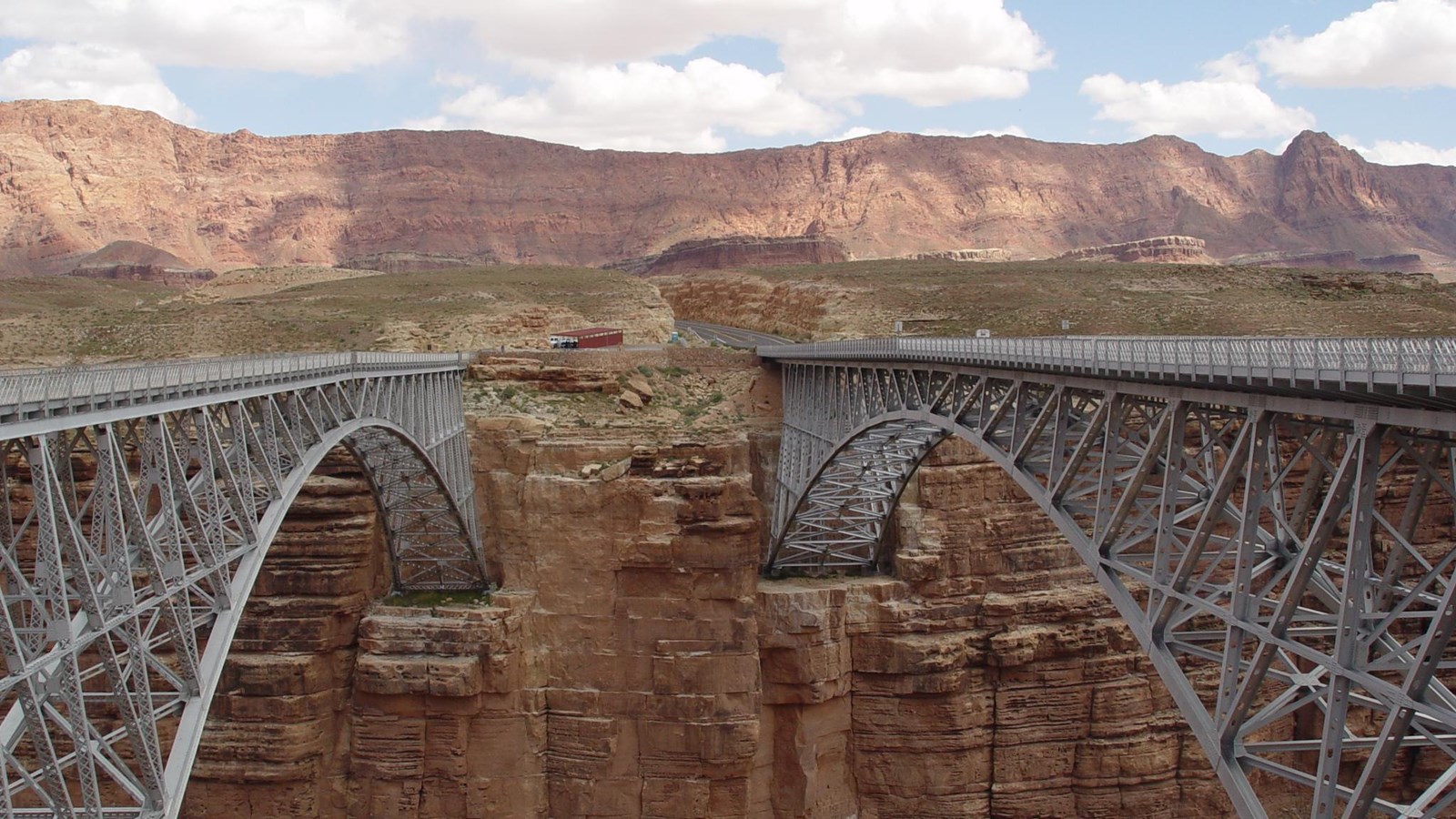This outdoor photograph captures a stunning canyon scene under a vibrant blue sky dotted with fluffy white clouds. Dominating the background is a towering, flat-topped red mountain that descends into sheer cliffs. Midground, two silver metal bridges arch gracefully over a yawning canyon, supported by intricate steel structures forming archways underneath. Both bridges converge towards the mountain in the background, with roads laid out on top. You can see a large truck, or possibly a car, making its way across the left bridge. In the foreground, patches of green grass add a touch of color, contrasting sharply with the earthy tones of the canyon walls and the metallic sheen of the bridges.